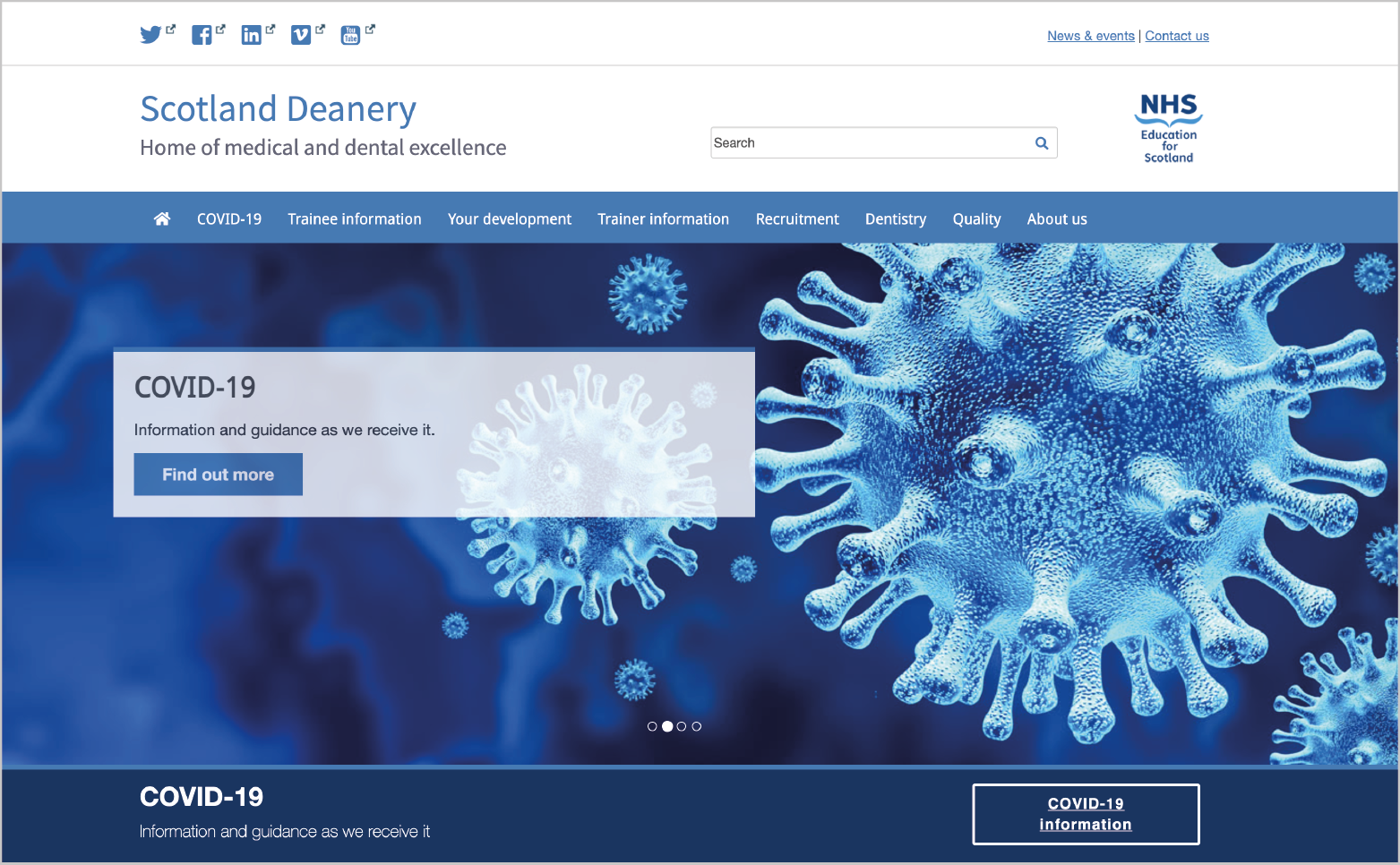The image is a screenshot of the homepage of the Scotland Deanery website, titled "Home of Medical and Dental Excellence." On the right side of the header, the NHS Education for Scotland logo is prominently displayed, attesting to its affiliation with the UK's National Health Service. The website's theme is predominantly blue and white, giving it a clean, professional appearance.

Central to the homepage is a large, eye-catching banner that focuses on the COVID-19 pandemic, with an image of the coronavirus. The banner provides essential information and guidance related to COVID-19, with a call-to-action button in blue that reads "Find out more." This suggests that the website offers timely updates and resources for managing the pandemic—a critical service during the height of the crisis.

The top left corner features social media icons for Twitter, Facebook, LinkedIn, Vimeo, and YouTube, indicating the site's active online presence and avenues for further engagement. At the top right, there are links for "News and Events" and "Contact Us," as well as a search bar for easy navigation.

Overall, the website appears to be a credible source for evidence-based advice, targeting medical and dental professionals in Scotland.